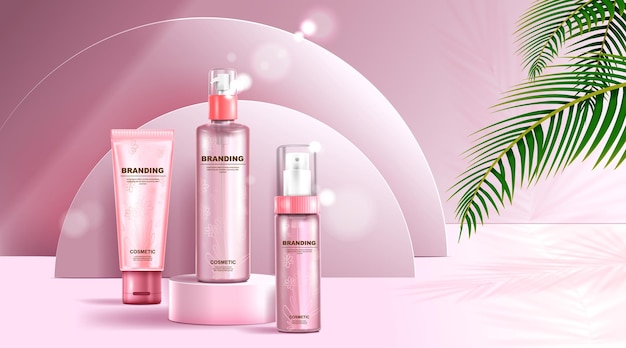The image depicts a stylish advertisement for cosmetic products, prominently featuring a trio of pink, metallic bottles set against a vibrant, computer-generated pink background. The background consists of two overlapping semicircles, resembling large plates, with lighting effects emanating from the right side. Adding to the tropical and modern aesthetic, palm fronds extend into the top right corner. The product lineup includes a lotion bottle on the left, a pump bottle taking center stage on a small pedestal, and a spray bottle on the right. Each bottle is adorned with nondescript text and the word "branding," with "cosmetic" inscribed at the bottom. This meticulously designed layout evokes a mod beach vibe, reminiscent of a high-end magazine spread, even though it features placeholder branding text.